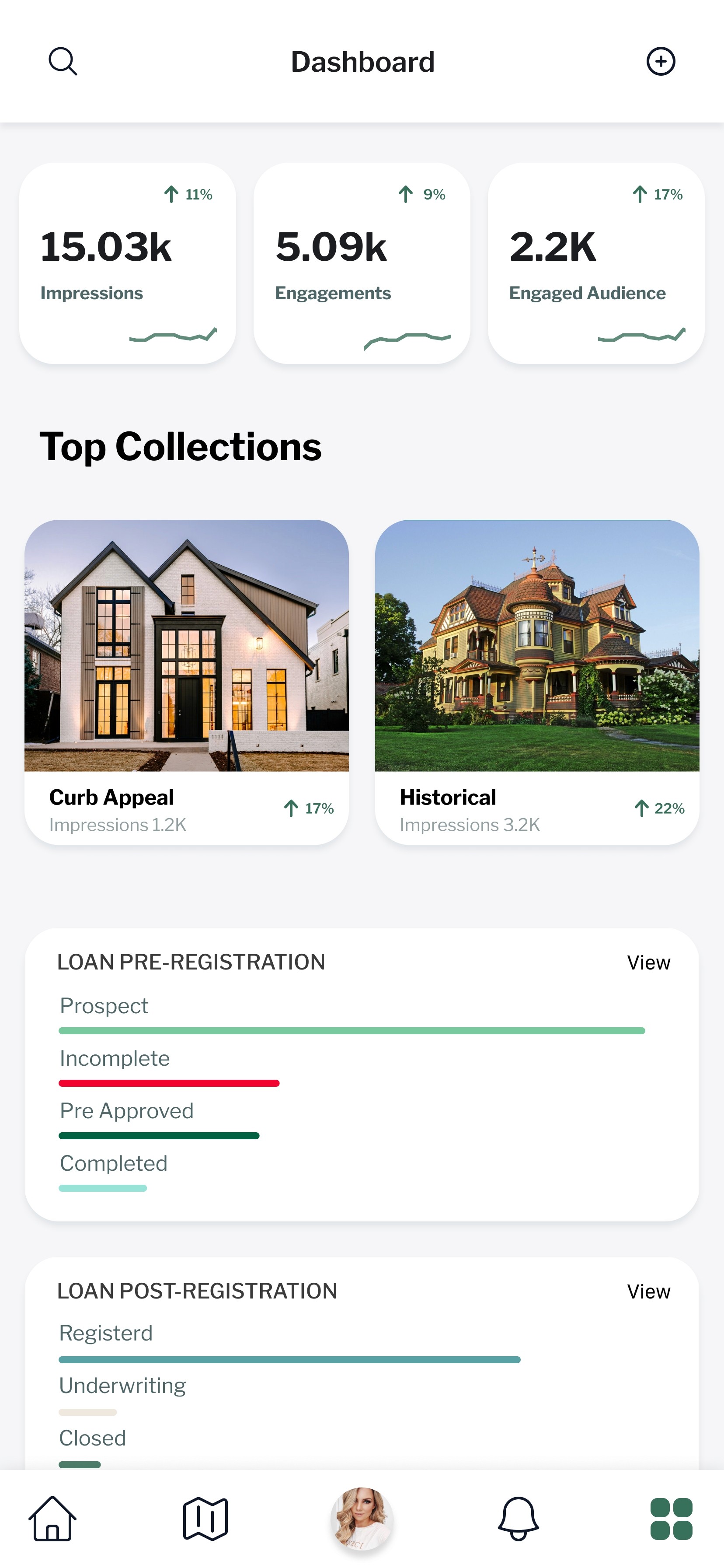A detailed and cleaned-up version of the provided voice caption could be:

---

**Real Estate Sales Dashboard**

The dashboard appears to be designed for real estate professionals or loan officers, providing various metrics and insights to track performance. The main screen displays several key statistics, including:

- **15,000 Impressions:** The number of times the listings or offers have been viewed.
- **5,009 Engagements:** The total interactions with the listings or offers.
- **2,002 Engaged Audience:** The number of unique users who actively engaged.
- **Performance Metrics:** Statistical data showing percentage changes, likely comparing month-to-month performance.

The dashboard includes several categorized data points:

- **Top Collections:** Details on the most popular listings or property categories.
- **Curb Appeal Impressions:** Visual appeal metrics for listed properties.
- **Historical Impressions:** Historical data on property views.
- **Loan Pre-Registration:** The stage before formal loan application.
- **Prospect:** Potential clients identified.
- **Incomplete:** Partially completed applications or leads not yet finalized.
- **Pre-Approved:** Applications that are pre-approved for loans.
- **Completed:** Successfully completed loan applications.
- **Loan Post Registration:** Stages following the initial loan registration.
- **Registered:** Clients formally registered in the system.
- **Underwriting:** Loans currently being reviewed.
- **Closed:** Finalized and approved deals.

Visual elements in the dashboard include an image of a house, a bell icon for notifications, a profile picture of presumably the user or agent, and a navigation menu at the bottom. This comprehensive tool likely assists real estate agents or loan officers to monitor and manage their sales and client interactions effectively.

---

This caption provides a clear, organized, and detailed description of the dashboard, highlighting its primary functions and features.